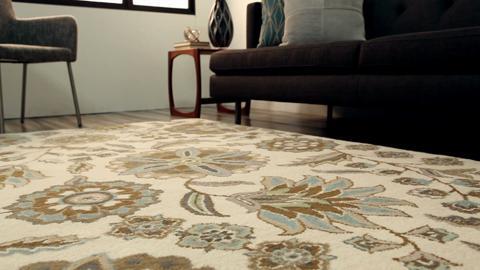In this image, we view a well-lit, modern living room predominantly featuring a light beige rug adorned with various floral patterns in shades of grey, brown, light blue, and deeper brown. The rug rests on a polished hardwood floor. To the right, there is a low, modern black couch fitted with throw pillows. A small cherry red wooden stool stands beside the couch, supporting a vase with a diagonal lattice design. In the backdrop, a contemporary coffee table holds a few books, positioned in front of the couch. Adjacent to the wall, another chair complements the overall décor. An edge of a window, just out of frame, allows natural light to flood the impeccably clean room, highlighting the elegant and cozy interior of this modern home.